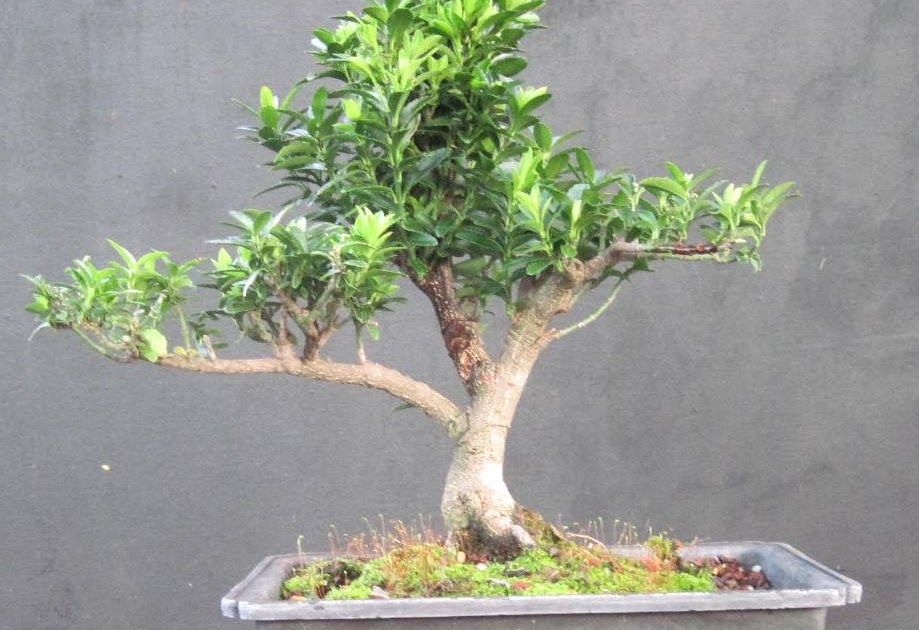This photograph captures a bonsai tree meticulously planted in a rectangular, concrete-like gray tray, occupying about 75% of the image's width at the bottom. The bonsai, resembling a miniature tree, features a small, V-shaped brown trunk with several branches—one notably long extending horizontally to the left, while others reach upward. The foliage showcases a mix of lush, vibrant green leaves, both light and dark. The base of the tree is surrounded by soil with patches of green moss and grass-like plants. The backdrop is a textured, medium gray concrete wall, adding a stark, minimalist contrast to the vividness of the bonsai.